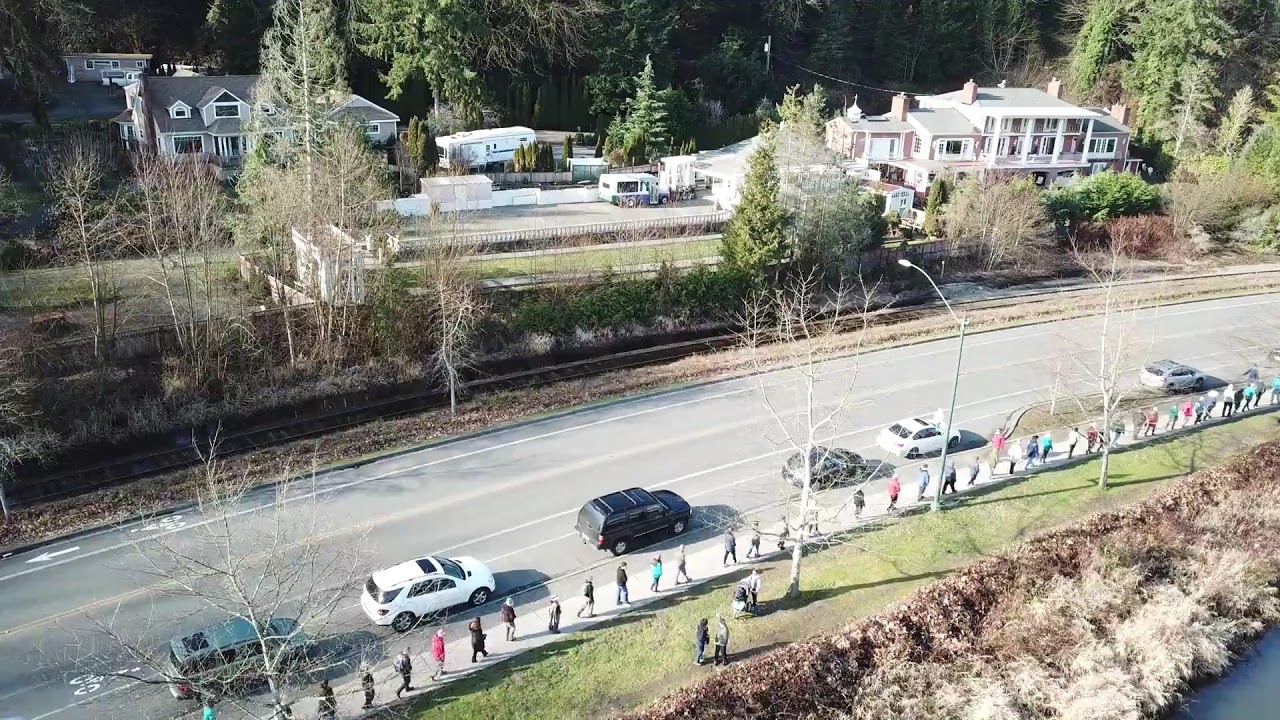The image displays an aerial view of a rural town nestled within a forested area during fall or winter, evident from the bare trees dotting the landscape. Central to the image is a road flanked by a long sidewalk bustling with around a hundred older pedestrians, some of whom carry backpacks. On the right side of the road, cars are parked closely together, while on the opposite side of the sidewalk, a patch of green grass stretches out before transitioning into dried brambles and herbage, culminating at the edge of a water body, possibly a lake. The presence of a railroad track runs parallel to the road, situated between the lush, bare, and evergreen trees framing the scene. Adjacent to the road, imposing brick and white-walled houses with grey roofs stand prominently in both the foreground and background, adding to the suburban feel. Further beyond, verdant forested hills rise, integrating the town seamlessly into its natural woodland surroundings.